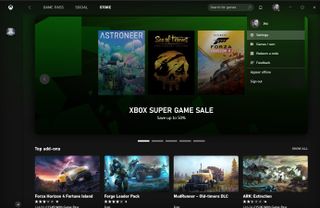The screenshot depicts the Xbox website, showcasing the "Xbox Super Game Sale" prominently in white text in the center. The page is designed against a black background, emphasizing the colorful and vibrant images of various games on sale. 

At the top of the page, there are five navigation tabs with the first one highlighted. The central banner of the webpage shows the text "Xbox Super Game Sale" with visuals that include the game "Astroneer," characterized by cloudy imagery and a faint skull motif. 

Beneath the main text, several game images are displayed in sections. The first highlighted game has indistinct text and visuals that possibly depict a waterway and rocks. To the right, there are six more sections featuring different games. One section shows vividly colorful and cloud-like graphics, while another section displays a character resembling a humanoid robot soldier with a military vehicle in the backdrop. Further right, an image of a semi-truck is visible, followed by an image of a barren wasteland.

The overall layout and design elements suggest that this is a promotional webpage dedicated to the Xbox "Super Game Sale," likely on the official Xbox website.